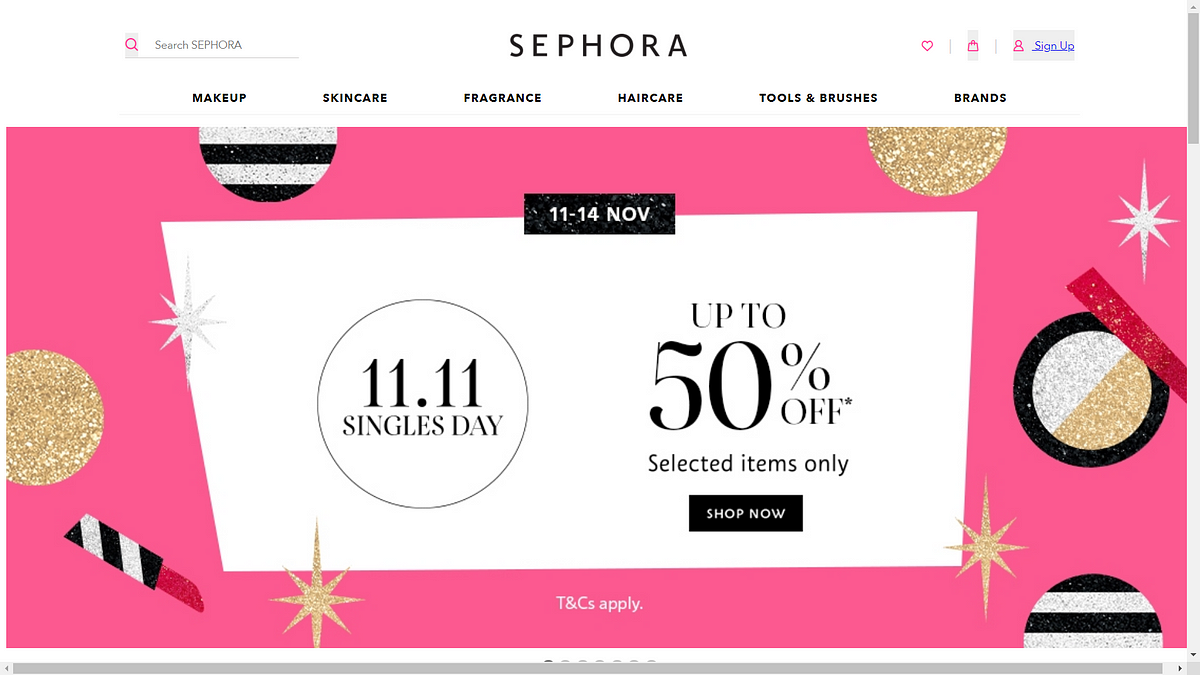This image is a detailed screenshot of a Sephora website. The layout is in landscape orientation, making it wider than it is long. In the upper left corner, there is a search bar labeled "Search Sephora." Centrally positioned is the headline “Sephora.” On the right side of the webpage, there are several icons: a heart symbol, a highlighted small box of unknown purpose, a profile picture icon, and a highlighted "Sign Up" link.

Beneath the headline, there is a navigation bar with several selections: Makeup, Skin Care, Fragrance, Hair Care, Tools & Brushes, and Brands. The main section of the website features a pink background with a scattering of various makeup items. There are several circular compacts containing what appears to be powder; one is open, revealing silver and gold colors, likely eyeshadows. Additionally, there is a lipstick tube with the lipstick extended.

Amidst the pink background, there is a prominent white box. At the top of this white box is a black banner displaying the dates "11-14 November." Below it, a circle denotes "11-11 Singles Day," alluding to November 11th being Singles Day. The text indicates “up to 50% off selected items only,” emblazoned across the white area. Below the discount information, a black “Shop Now” banner invites users to take action. Further down, the text "T&Cs apply" indicates that terms and conditions apply.

The image also features decorative gold and silver starburst emblems scattered around, adding to the festive and promotional feel of the webpage.